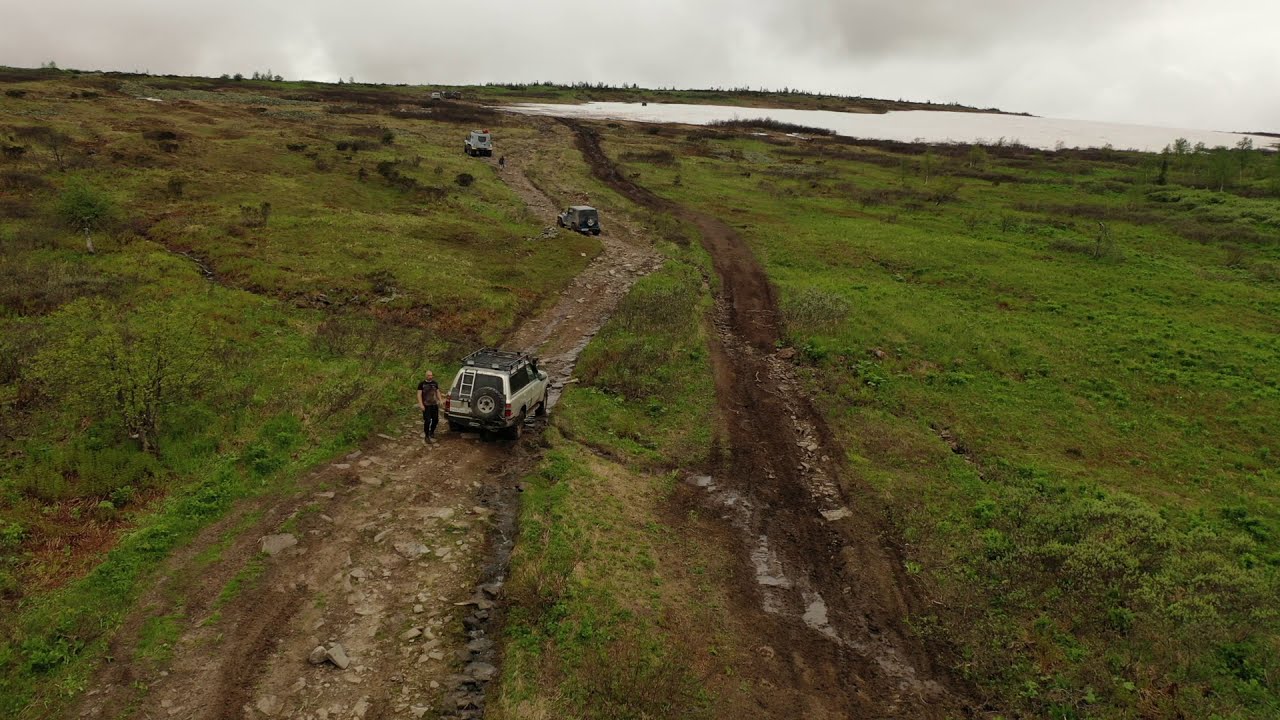The aerial photograph captures a scenic, somewhat undulating landscape that seems to be part of a European moor. Dominated by lush, grassy terrain interspersed with small rises and dips, the image prominently features two winding, muddy, and rocky off-road trails. The more pronounced left trail, tan and light brown in color, hosts three SUV-like cars, possibly Jeeps, making their way upwards toward a large body of water positioned in the upper center to right of the frame. The right trail, appearing wetter and darker, shows signs of erosion with pockets of water, indicative of past wear and tear. Gray, cloudy skies cover the scene, adding a somber tone. On the leftmost trail, a man clad in all black with graphic designs on his shirt stands next to the last car closest to the camera, adding a human element to the rugged terrain. The landscape is dotted with small trees and various low-level vegetation, painting a picturesque outdoor adventure setting.